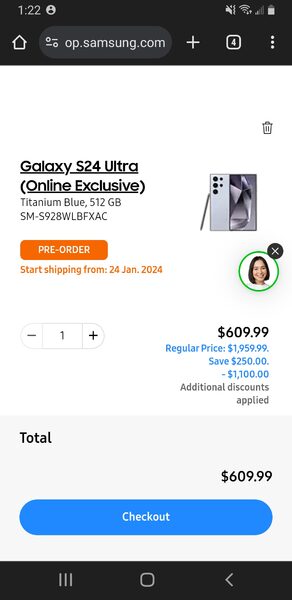This screenshot captures the checkout page on the Samsung website for the pre-order of the Galaxy S24 Ultra. At the top, the screen features a black header. On the far left of the header, there's a house icon. Next to this, a search bar displays the URL "Samsung.com," followed by a plus sign for adding another browser tab. Proceeding further right, there's a square icon indicating that four tabs are currently open.

Below the black header, the website body displays a white background. On the left side, the product details are prominently shown: "Galaxy S24 Ultra (Online Exclusive)." Beneath this, detailed product specifications are listed in smaller font: "Titanium Blue, 512GB," followed by the serial number. An orange "Pre-order" button is displayed, alongside information hinting that shipping will commence from January 24, 2024.

To the right of these details, there is a small image depicting the phone’s front and back views with a stylus leaning against it. Further right, in the central part of the screen, a circular chat bubble displaying a woman's head on a white background appears, suggesting a live chat option. An "X" icon allows for closing this chat bubble.

At the bottom of the screenshot, a gray box contains the final checkout summary. The total price is listed on the top left and again on the bottom right, quoted at $609.99. To complete the purchase, a prominent blue "Checkout" button is fixed at the bottom right corner of the gray box.